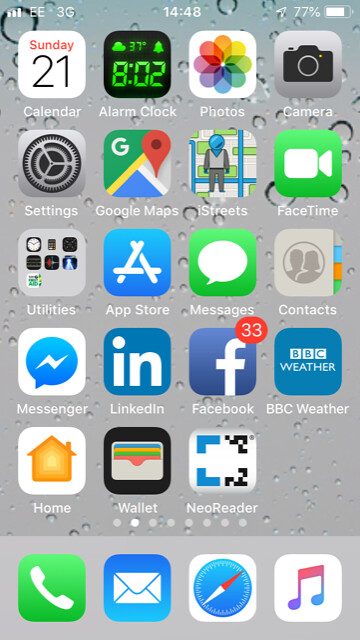Screenshot of a smartphone home screen featuring a variety of application icons: At the top, the "Calendar" icon displays "Sunday 21." The "Alarm Clock" icon shows the time "8:02" and the temperature "37 degrees." The "Photos" icon features a rainbow-colored image stack, and the "Camera" icon depicts a black camera body. The "Settings" icon is represented by multiple gear shapes.

"Google Maps" is shown with the letter "G" in the upper left corner, a red location pointer on a green, blue, and gray map layout. "iStreets" displays a figure standing over a street map. "FaceTime" is represented with a green background and a white camera icon. The "Utilities" folder contains various smaller icons, indicating a collection of apps.

Other visible apps include "App Store," with a stylized 'A' made of three lines, "Messages" depicted with a green background and a white speech bubble, and "Contacts" illustrated by a silhouetted image of a man and a woman within a circle. "Messenger" shows a lightning bolt inside a speech dialog box, "LinkedIn" features a blue background with the lowercase letters 'in,' and "Facebook" includes a lowercase 'f' on a blue background. 

"BBC Weather" is represented by the BBC logo and the word 'Weather' on a blue backdrop. "Home" illustrates a house icon, and "Wallet" displays a multicolored wallet. "Neo Reader" does not have a detailed visual description. 

At the bottom, the screen includes icons for a phone, messages, a compass, and music notes.